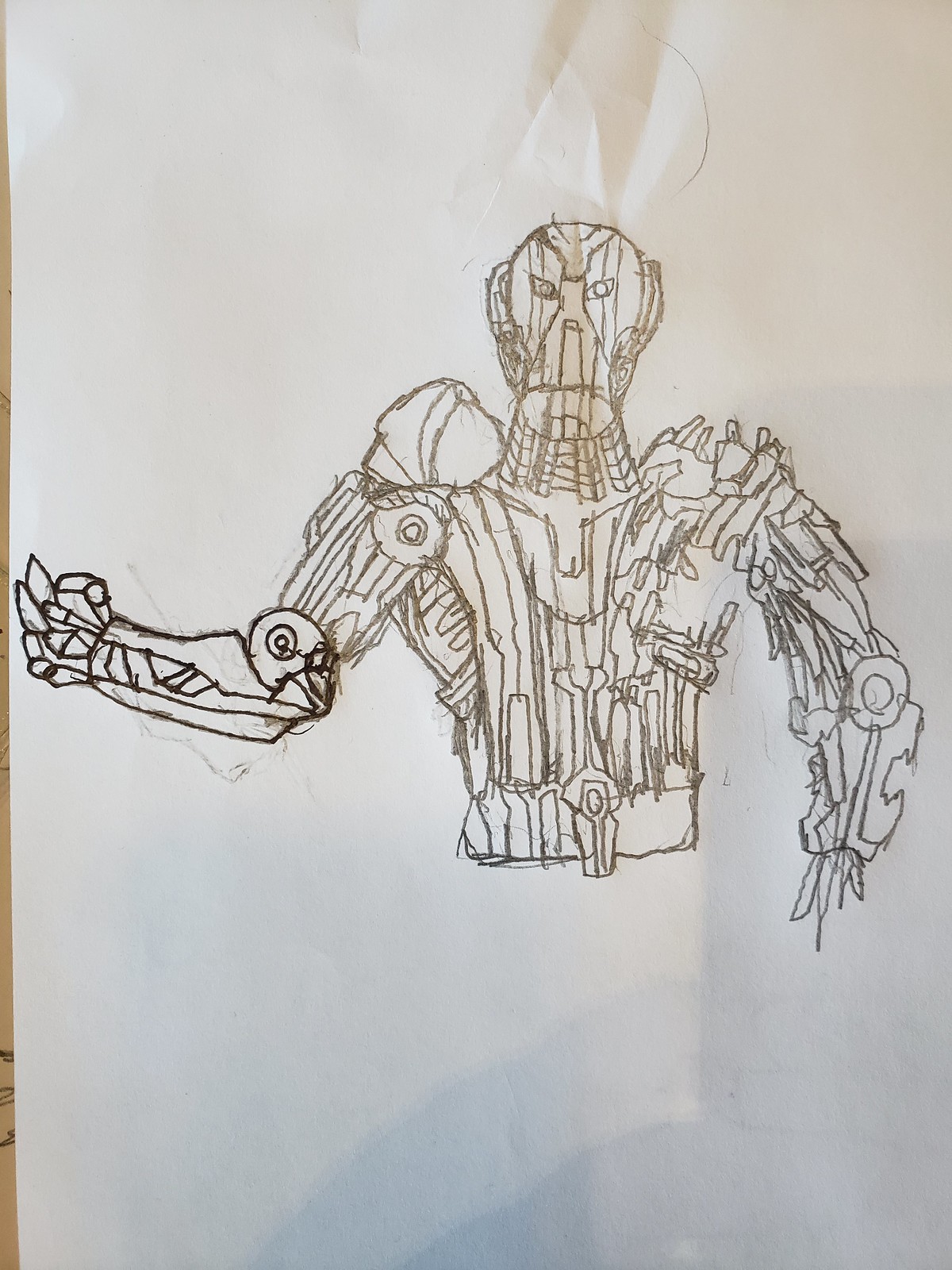The image depicts a detailed drawing of a humanoid, possibly reptilian alien warrior, on a slightly wrinkled piece of white computer paper with areas shaded in gray. The artist seems to have used a fine-point marker for enhanced precision. The alien's head has a generally human shape but features distinctly non-human characteristics: the eyes slant upwards at the outer corners, reminiscent of reptilian eyes, and the nose has an unusual, reptile-like structure. The face is marked with prominent lines, and the ears, if they are ears, appear flat against the head. The creature has a wide neck leading into ornate armor, which is visible down to the waist. The armor is intricate, with exaggerated shoulder pads; the right shoulder pad is notably larger than the left, which seems incomplete or different in design. The alien's right arm, from the viewer's left perspective, has a mechanical, jointed elbow featuring a central circle with two nested smaller circles. The elbow is bent, with the hand outstretched, showing non-human, mechanical fingers that end in points.